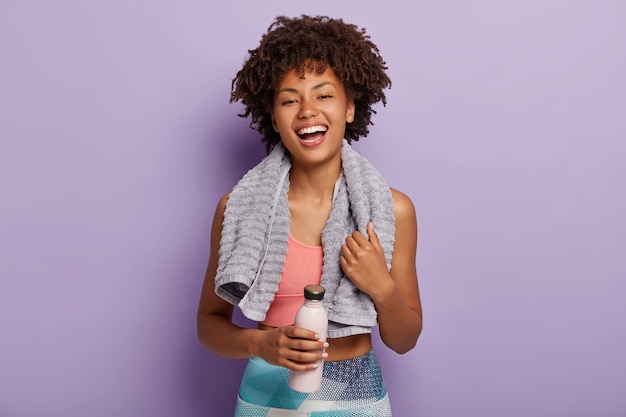A vibrant and detailed photograph captures an African-American girl with stunning, curly twists in her hair, standing confidently in front of a lavender purple wall, which gives the image a studio-like clarity and brightness. She radiates joy with a wide, beaming smile, her expression of happiness filling the space. Dressed in a salmon-colored crop top designed for exercise, paired with blue and light blue bike shorts adorned with geometrical shapes and hints of purple, she embodies a lively, athletic spirit. Draped casually around her neck is a fluffy gray towel, suggesting she’s either just finished a vigorous workout or is about to start one. In her right hand, she holds a sleek white water bottle with a black top, and her left hand rests lightly on the towel, enhancing the relaxed yet energized vibe of the scene.